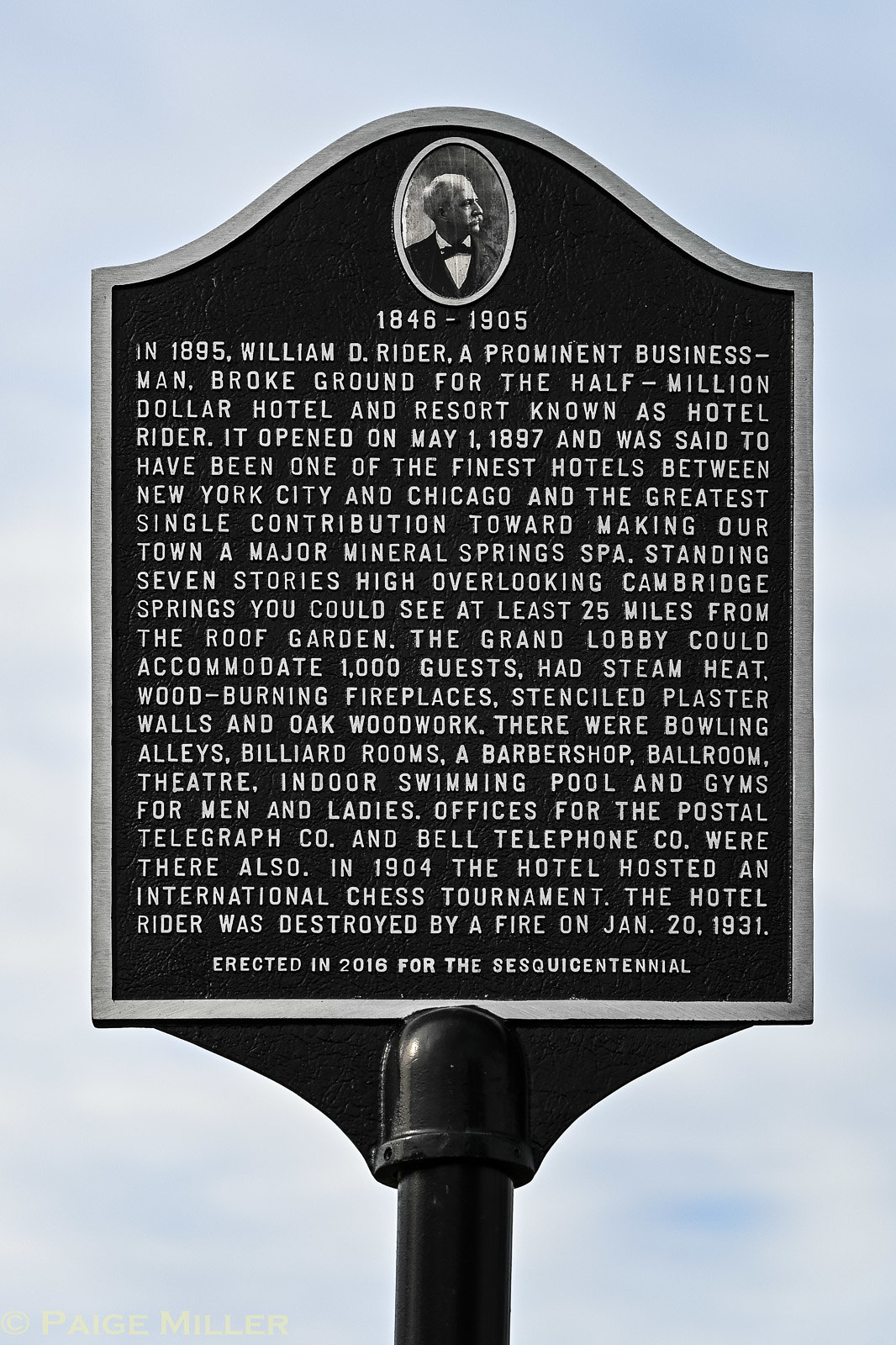The image features an elegant, historical marker set against a backdrop of blue sky and white clouds. The black rectangular placard, mounted on a black metallic pole, has a slightly triangular bottom connecting to the pole and a rounded top. The top part of the marker houses an oval black-and-white side portrait of an older man with grey hair, donned in a black jacket, black bow tie, and white button-up shirt. Beneath the portrait, the inscription reads "1846-1905" in white text. The sign commemorates William D. Ryder, a prominent businessman who, in 1895, began the construction of the half-million-dollar Hotel Ryder. Opening its doors on May 1, 1897, the hotel was hailed as one of the finest between New York City and Chicago.

Further inscriptions describe the hotel, which stood seven stories high and overlooked Cambridge Springs. From its roof garden, guests could view up to 25 miles, and its grand lobby could accommodate a thousand guests. The establishment featured steam heat, wood-burning fireplaces, stenciled plastered walls, and oak woodwork. Amenities included a bowling alley, billiard rooms, a barbershop, a ballroom, a theater, an indoor swimming pool, and separate gyms for men and women. Essential services like the Postal, Telegraph Company, and Bell Telephone Company were also present, marking the Hotel Ryder as a significant contributor to making the town a notable mineral spring spa. The marker itself was erected in 2016, celebrating the centennial and testament to the hotel's lasting historical impact.